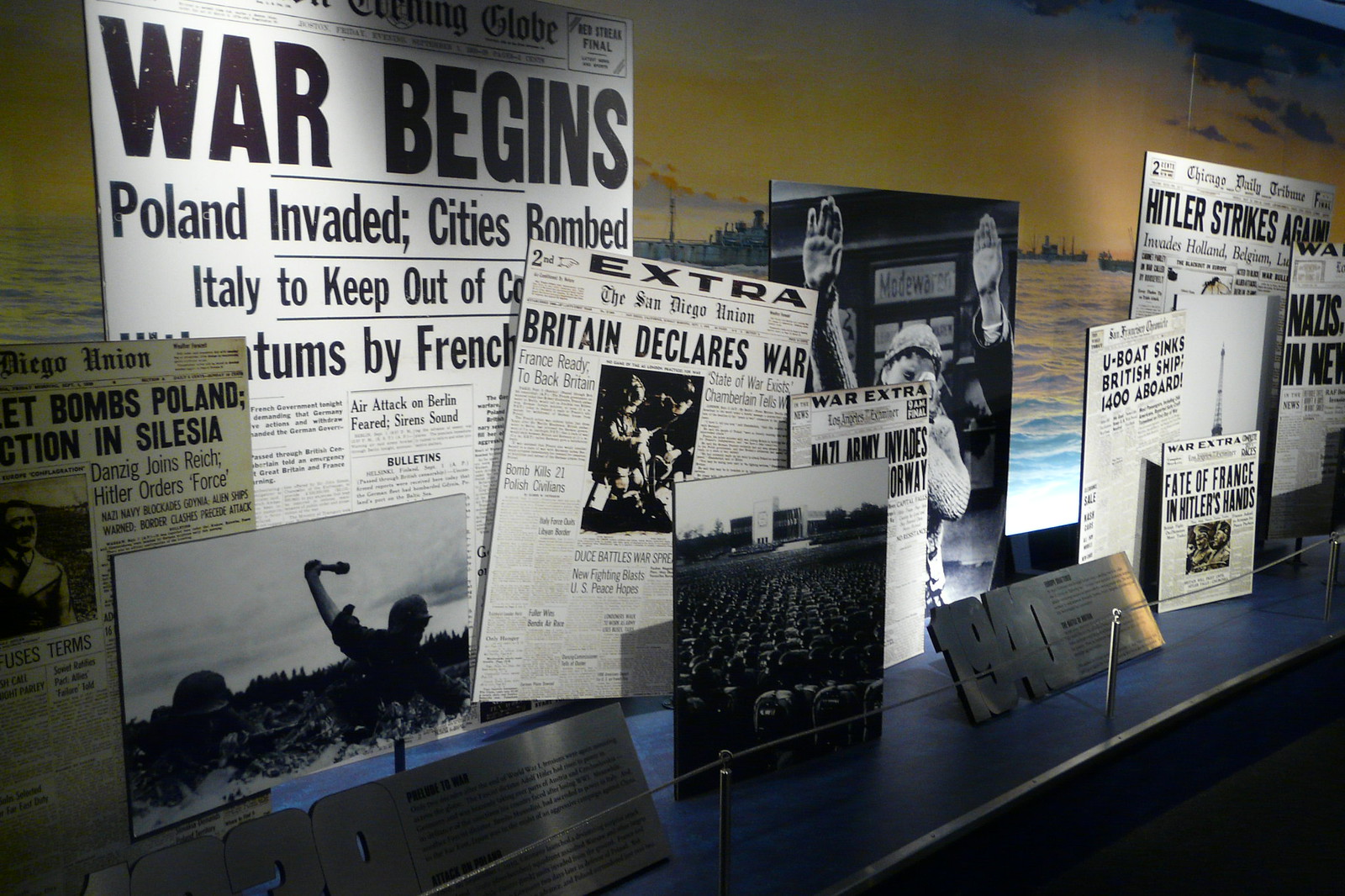This photograph showcases a detailed and somber museum exhibit dedicated to World War II. Dominating the scene are numerous black-and-white newspaper headlines and war propaganda posters displayed on sturdy backings. Each headline chronicles pivotal moments: "War Begins: Poland Invaded," "Cities Bombed," "Italy to Keep Out," "Britain Declares War," and "U-boat Sinks British Ships: 1,400 Aboard." Another stark headline reads, "Fate of France in Hitler's Hands," with yet another pronouncing "Hitler Strikes Again." Among the posters, there are also black-and-white photos, including one showing children making the Hitler salute and another depicting a large crowd. The exhibit is roped off to prevent contact from museum-goers, all set in a relatively dark room which enhances the gravity of the historical content. A subtle touch of color in the background, resembling a painted sunset over a sea, adds a contrasting softness to this otherwise monochromatic and impactful display.